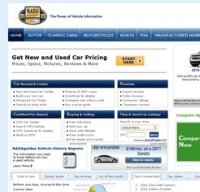The screenshot is notably small and blurry, rendering most of its text illegible. The only discernible phrase reads "get new and used car pricing." A highly blurry image of a car is visible near the bottom of the screenshot. The car appears to be a four-door silver Hyundai sedan, parked with its front facing towards the right. Despite close examination, no other people, animals, plants, buildings, motorcycles, bicycles, airplanes, helicopters, trains, boats, billboards, or flags can be identified in this image due to its poor quality.